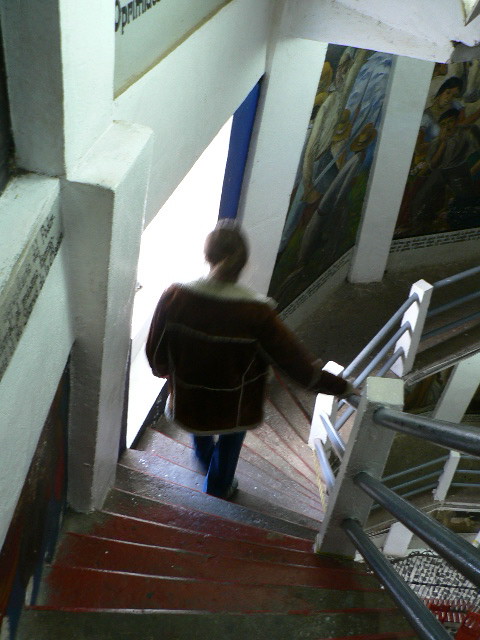In this image, a woman with a ponytail, wearing a brown jacket with a white collar and blue jeans, is walking down a steep, possibly spiral staircase that appears indoors. The scene is slightly blurred, adding a soft focus effect. The stairs themselves are wooden and painted in shades of red, green, and possibly brown. She has her right hand on a gray railing that runs along the right side, consisting of metal poles and pillars. The staircase curves to the right as it descends, and the steps are very close together, emphasizing the tightness of the staircase.

The environment around her resembles a museum or cathedral, indicated by the artwork on the predominantly white walls. These paintings, which appear to be from the 1st to 5th centuries, are positioned between white pillars and sections of the wall. The lighting suggests it is daytime, with natural light streaming through a nearby window. Additionally, there is some written text on the left side of the wall. The right-hand side wall features a mix of black, white, and red sections, adding a contrasting element to the scene.